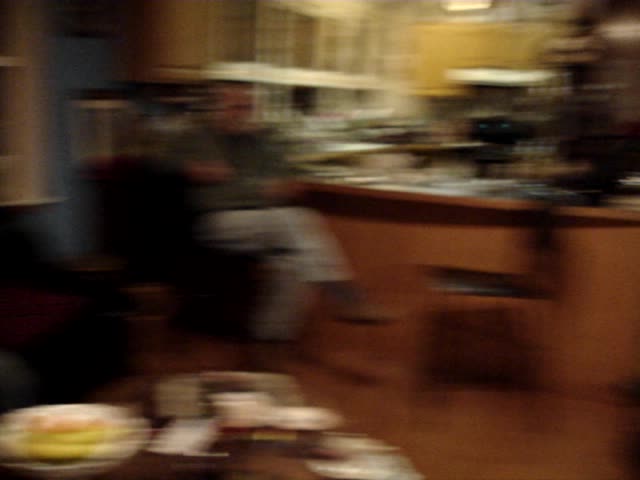A slightly out-of-focus image captures a man seated at a kitchen island, viewed from the left. He is perched on a stool, legs crossed, and is dressed in light blue pants, brown boots, and a long-sleeved green shirt. The kitchen in the background features tan cabinets lining the back wall. To the man's right, another brown chair faces him directly. In the bottom left corner of the frame, part of a round dining table is visible, adorned with food and a glass or plastic container. Towards the bottom right of the table, a few rounded containers can also be seen.